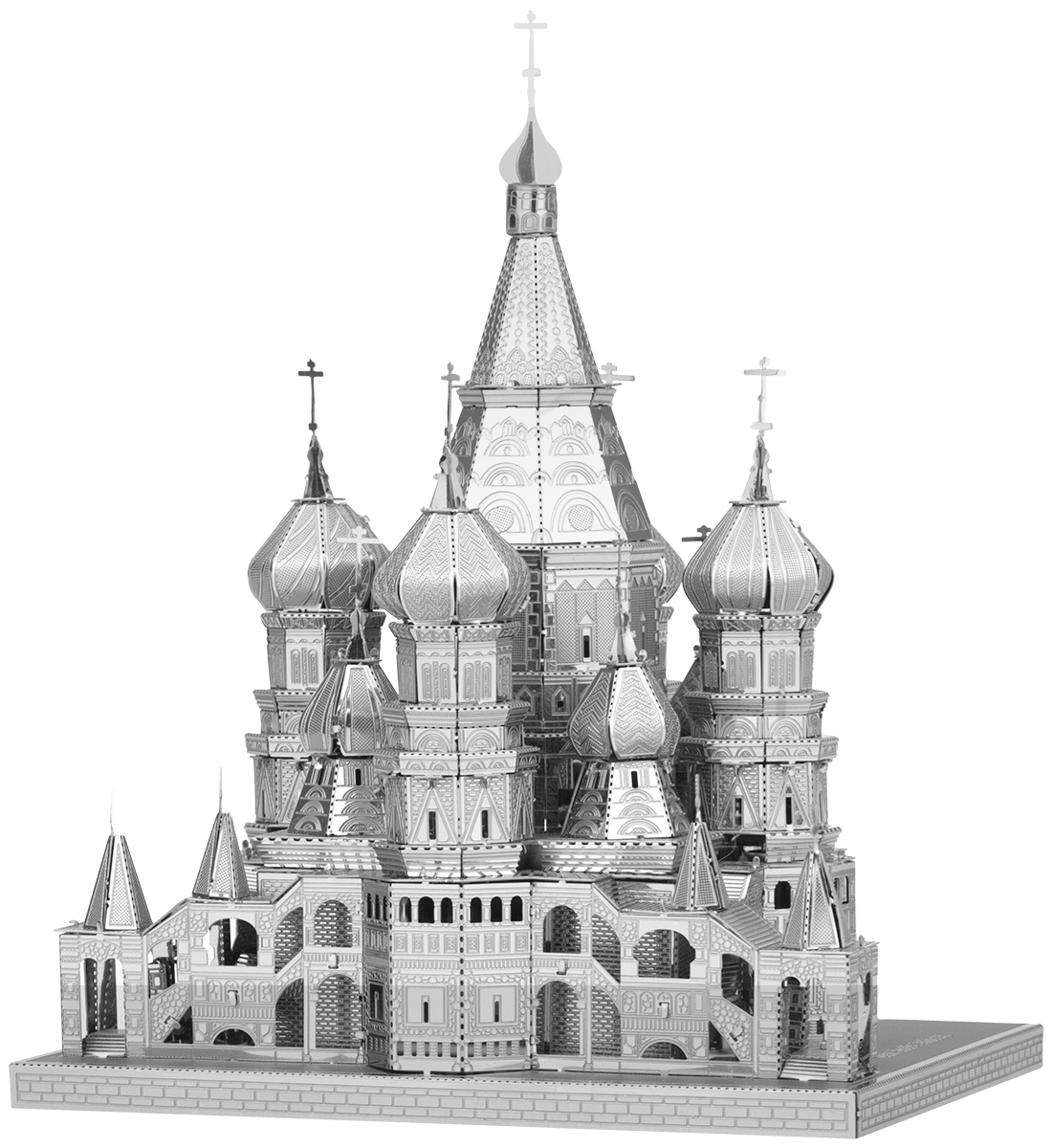This vertically aligned, black-and-white image portrays an intricately detailed sculpture resembling a Russian Orthodox cathedral. The structure, appearing to be made of metal, displays fine craftsmanship with perforated dotted lines along its seams, suggesting it could be assembled like a model kit. The robust base, which exhibits an etched wood grain texture and a brick pattern, provides a solid foundation for the grand cathedral above.

A towering central turret, hexagonal in shape with a pointed dome, dominates the scene. Flanking this main tower are four smaller turrets, each topped with rounded domes and a cross. The meticulous design includes very tall double doors at the front entrance and enclosed stairways on either side leading to the second level. The entire sculpture exudes a sense of historical and architectural richness, evoking the grandeur of a meticulously crafted cathedral model.